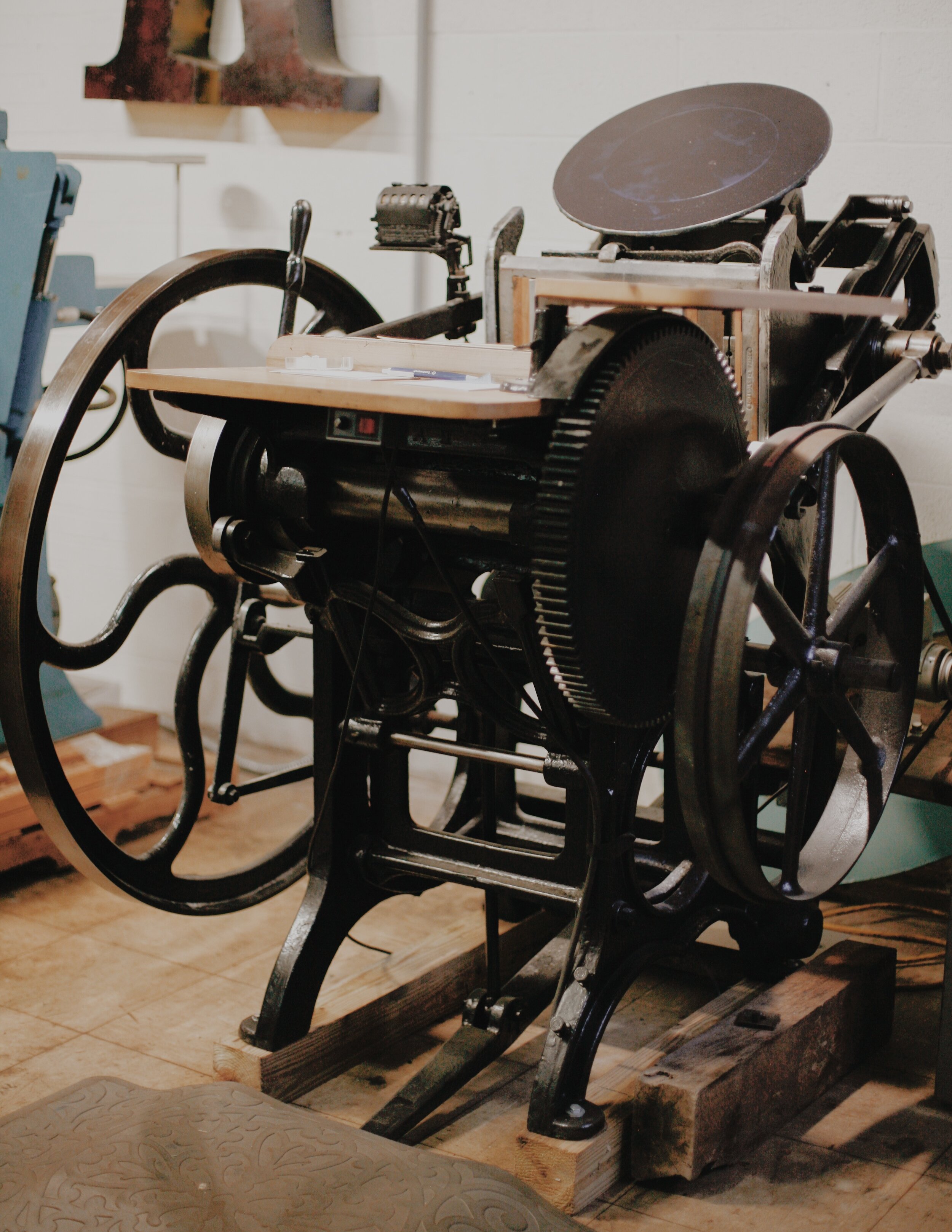The image depicts an antiquated printing machine, potentially from the early days of mechanical printing technology. The machine features two large wagon-style wheels, indicative of its considerable age. On one side, there is a notable brown metal plate, while the opposite side houses a meticulously arranged tray. The machine's operations appear to be managed by a prominent lever, connected to a dark brown spindle with ridged detailing. This entire apparatus is set upon a rustic, well-worn wooden base, resting on a matching wooden floor, suggesting its age and historical significance. The setting seems to be a museum, reinforced by the presence of another light blue piece of machinery in close proximity, possibly an exhibit companion. Above this secondary machine, a letter, likely an 'A', is partially visible, hinting at signage or additional context for museum visitors.